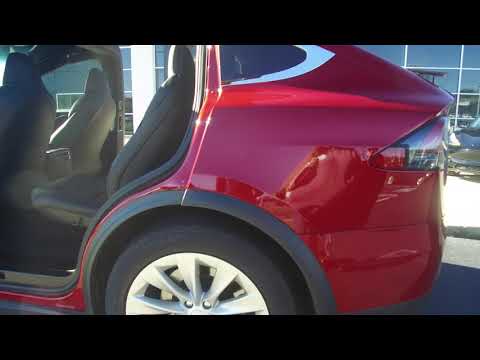The image captures a reflective deep red compact sedan, prominently viewed from the left rear side. Both rear doors of the four-door car are open, offering a clear view into its interior, which features dark gray cloth bucket seats. The vehicle sports black tires with metallic silver-colored hubcaps. Noteworthy in the background is a white-framed building with numerous windows, reminiscent of a dealership or office space, reflecting in the car's shiny surface. The scene includes a brightly lit sidewalk and asphalt ground, further emphasizing the vehicle's presence.